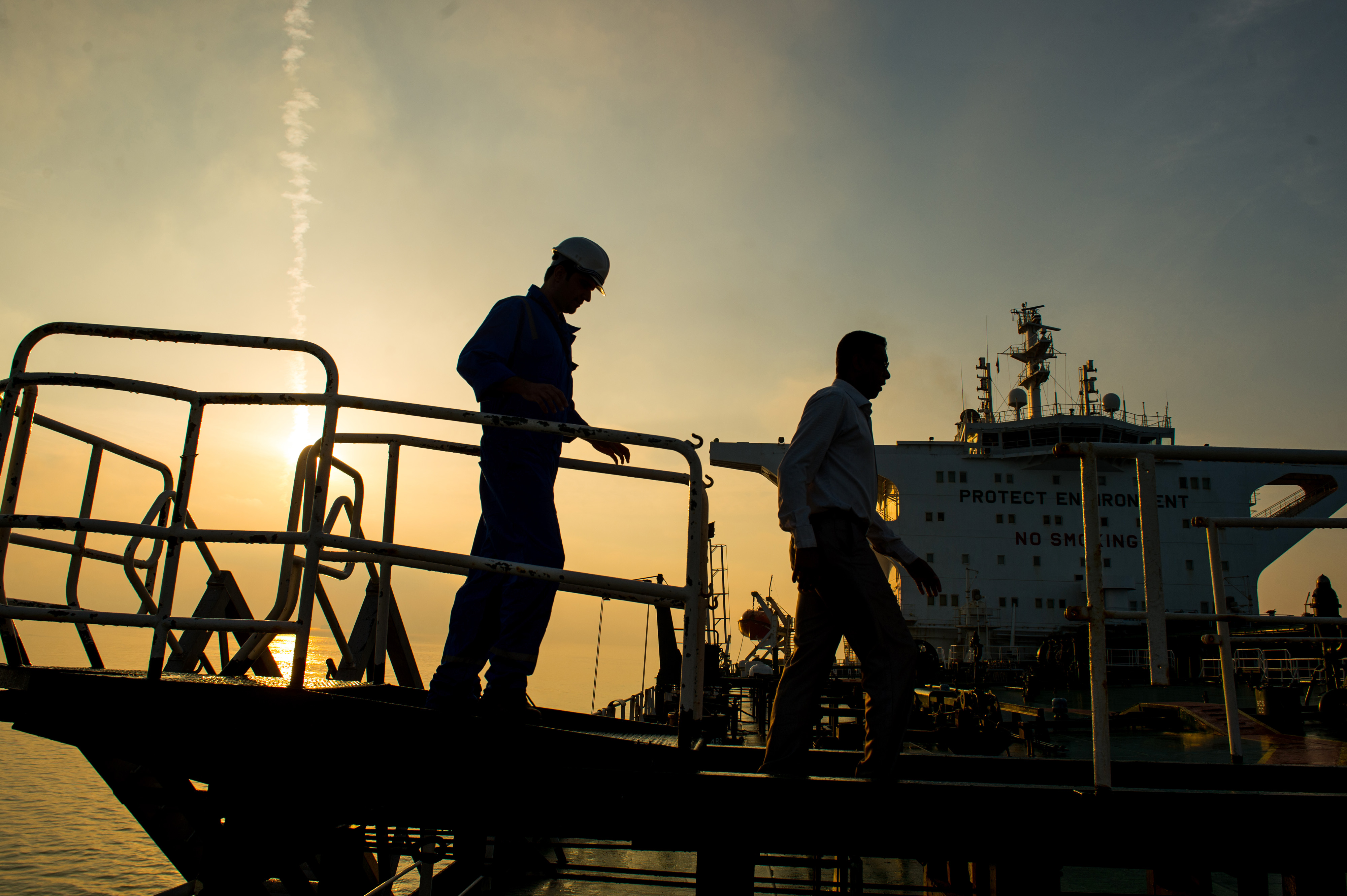The image depicts two silhouetted men walking down a grated plank toward the right side of the frame, likely at either sunrise or sunset, given the orange and pink hues reflecting off the water. The man in the back wears a hard hat and a long-sleeved shirt and pants, while the man in front is dressed in a white long-sleeved shirt and pants. They seem to be exiting a large work ship, possibly an oil tanker, identifiable by its towering structure with railings, cranes, and antenna-equipped bridge visible in the background. The ship prominently displays the messages "Protect Environment" and "No Smoking." The sky above is a vibrant mix of blue and white clouds, with the sun casting a starburst appearance as it grazes the horizon near the left-hand corner of the image.